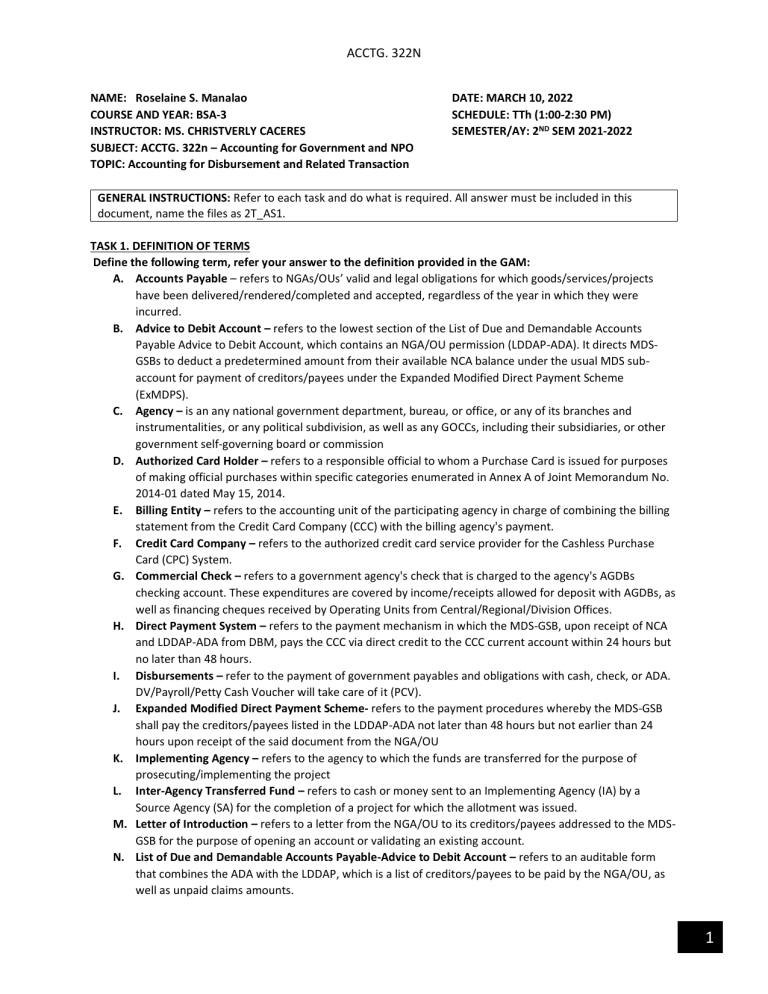Screenshot of Rosalene S. Manalow's coursework details for Accounting 322N

The image features a comprehensive screenshot of Rosalene S. Manalow's coursework for the accounting course "Accounting for Government and Non-Profit Organizations," specifically covering the topic "Accounting for Disbursement and Related Transactions." The details of the course are as follows:

- **Course Year & Section**: BSA 3
- **Instructor**: Ms. Christopher Lee Caceres
- **Course Date**: March 10, 2022
- **Schedule**: Tuesdays and Thursdays from 1:00 PM to 2:30 PM
- **Semester & Academic Year**: Second semester of 2021-2022

**General Instructions**:
- Refer to each task and perform the required actions.
- All answers must be included in the provided document.
- Name the files as "2T_AS1."

**Tasks**:
1. **Definition of Terms**: The document lists various accounting terms that need to be defined according to the Government Accounting Manual (GAM):
   - Debt Accounts Payable
   - Advice to Debt Account Agency
   - Authorized Cardholder
   - Billing Entry
   - Credit Card Company
   - Commercial Check
   - Direct Payment System
   - Disbursements Expanded
   - Modified Direct Payment Scheme
   - Implementing Agency
   - Inter-Agency Transfer Fund
   - Letter of Introduction
   - List of Due and Demandable Accounts Payable

The definitions appear to be partially completed. Despite a minor grammatical error in the instruction (using "answer" instead of "answers"), the coursework primarily focuses on detailed accounting terminologies and processes relevant to governmental and non-profit organizations.